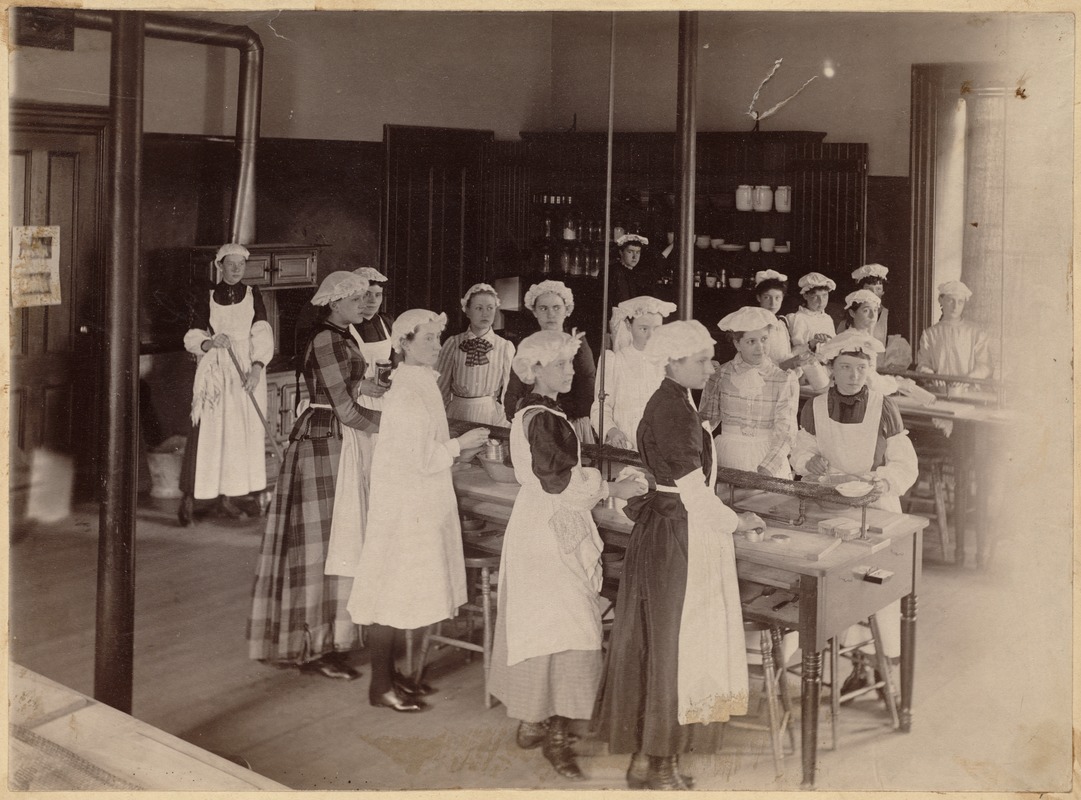This is an old, sepia-toned photograph depicting a group of sixteen women, likely workers or maids, engaged in a task that appears to involve baking or working in a factory. The image is in black and white but has a rusty, dark brown hue instead of pure black and gray. The women are all wearing a uniform consisting of white caps resembling shower caps, thick white aprons over stark and floor-length dark dresses, and lace-up black boots. Their attire suggests a historical context where such clothing and headgear were common among female workers. Notably, one woman stands apart on the left side of the photo, holding a mop, indicative of her role as a cleaner. In the background, there is a shelf filled with various bottles and jars, adding to the ambiance of a work environment. All the women are looking towards something or someone on the right side out of the frame, further hinting at their engagement in a shared task or receiving instruction.